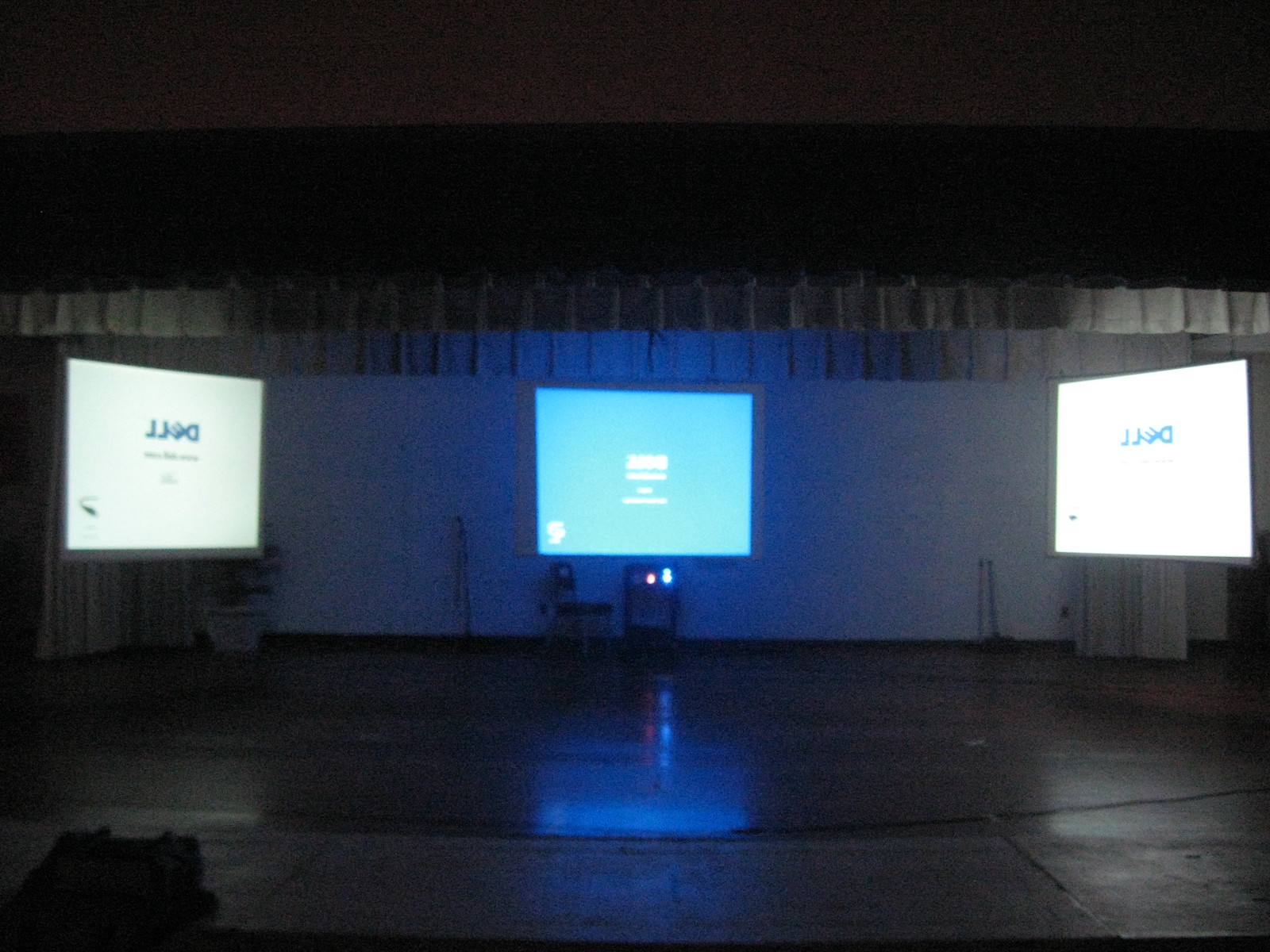The image depicts a dimly lit stage or auditorium with three large TV screens positioned towards the back wall. The screens are symmetrically arranged with one in the center and the other two flanking it on either side. The central screen has a light blue background with white text, likely the Dell logo, although it's not entirely legible. The screens on the left and right have a white background with a blue Dell logo prominently displayed. The floor below the screens is wooden and reflects the colors of the screens. Additional details include a black wall and mostly white curtains in the background. There is a chair beneath the central screen, a table with a lamp, and a plant in a white pot near the left screen. Additionally, there appears to be a black bag lying on the wooden floor in the lower-left corner of the image.